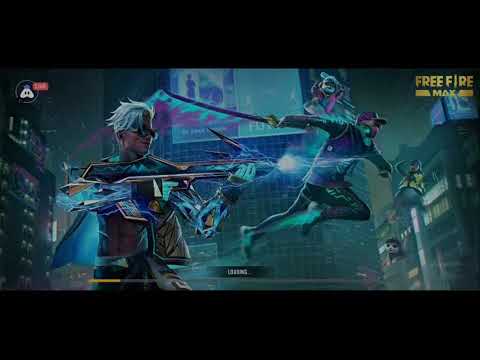This is a detailed screenshot from the loading screen of a video game titled "Free Fire Max". The image has black letterbox bars on the top and bottom, occupying approximately 20% of the total height. Central to the scene are two characters engaged in a cyberpunk-styled battle set in a futuristic cityscape with skyscrapers and large digital screens in the background. 

One character, situated on the left, is a young male with white spiky hair, wearing blue reflective sunglasses, an open jacket that reveals his chest, and a combination of futuristic attire. He is firing a gun that shoots a blue energy beam. On the right, another character is mid-air, sporting a black jacket, black pants, headphones, and a purple hat. This individual is equipped with a long, glowing katana sword that leaves a vibrant teal energy streak, with a similar blue trail emanating from his boots, suggesting rapid movement or possibly a jump.

In the upper right corner of the image, the text "Free Fire Max" is clearly visible. Beneath it is a control interface that seems to display a score or game status. The entire image appears slightly low-resolution with noticeable artifacts, and positioned in the middle is a gray bar with a yellow segment on the left, labeled "loading." The scene captures an intense moment of battle, showcasing a mix of futuristic weaponry and dynamic action.